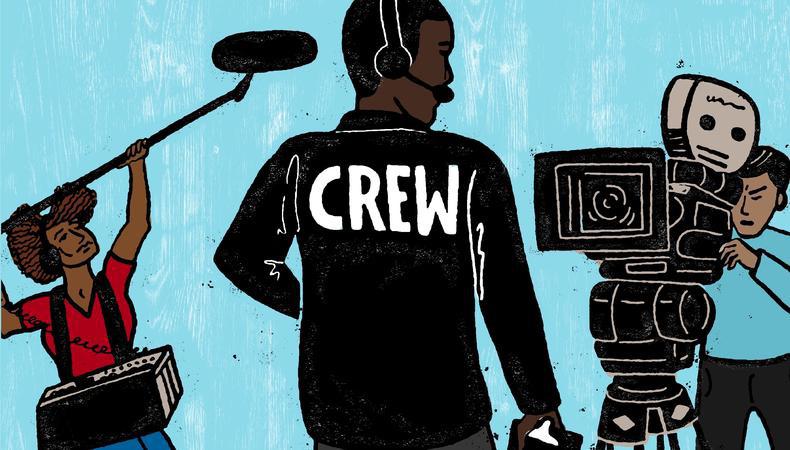In this vibrant cartoon painting of a film or news crew set against a textured blue backdrop with white smudges, the scene unfolds with meticulous detail. Central to the image is a black individual, facing away from the viewer, dressed in a long-sleeved black jacket boldly labeled "CREW" on the back. They are equipped with a headset, complete with earmuffs and a mouthpiece, and are holding a clipboard in their right hand. Their head is turned to the right, revealing their profile.

To the left of the central figure stands a woman with voluminous, Afro-ish brown curly hair, partially parted by the long oval-shaped black boom microphone she holds aloft on a large metal stick. She is dressed in a short-sleeve red shirt and blue pants, and slung over her shoulders are suspenders connected to a black box with dials, central to her role in sound management. She also wears headphones, intensifying her focus on capturing the perfect audio.

On the right side of the image, a racially ambiguous man operates a large professional camera, resembling an old reel-to-reel. He wears a long-sleeved blue shirt that blends with the background and dark pants. With one eye pressed against the camera’s eyepiece, he ensures the shot is perfectly framed as the camera, larger than him due to perspective, stands on a tripod, ready to record the scene.

The harmonious depiction of a diverse crew dedicated to their roles and responsibilities hints at a collaborative and inclusive filmmaking environment.